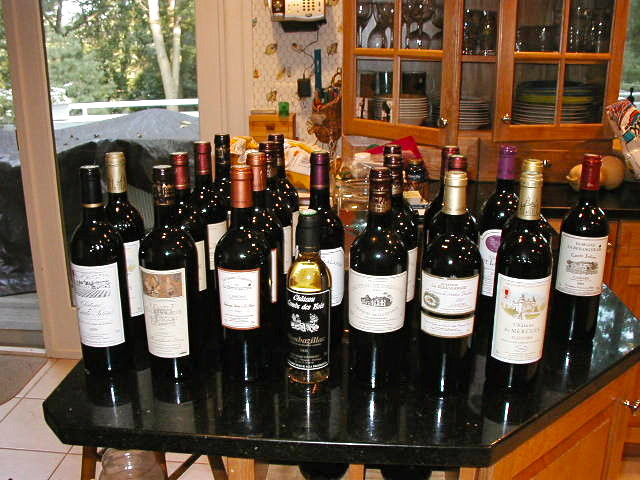The photograph showcases a kitchen with a black marble peninsula countertop, the focus of which is nearly two dozen wine bottles displayed in rows. Primarily dark-labeled, these bottles are accompanied by an amber-colored bottle in the center of the front row. The backdrop reveals an upper cabinet with glass doors, housing neatly stacked plates, wine glasses, and other dishes. Also visible in the kitchen are a bag of chips and some onions on the counter, along with a wall-mounted cordless phone receiver base. The kitchen leads to an outdoor area through a sliding glass door that frames a serene view of birch trees and evergreens.